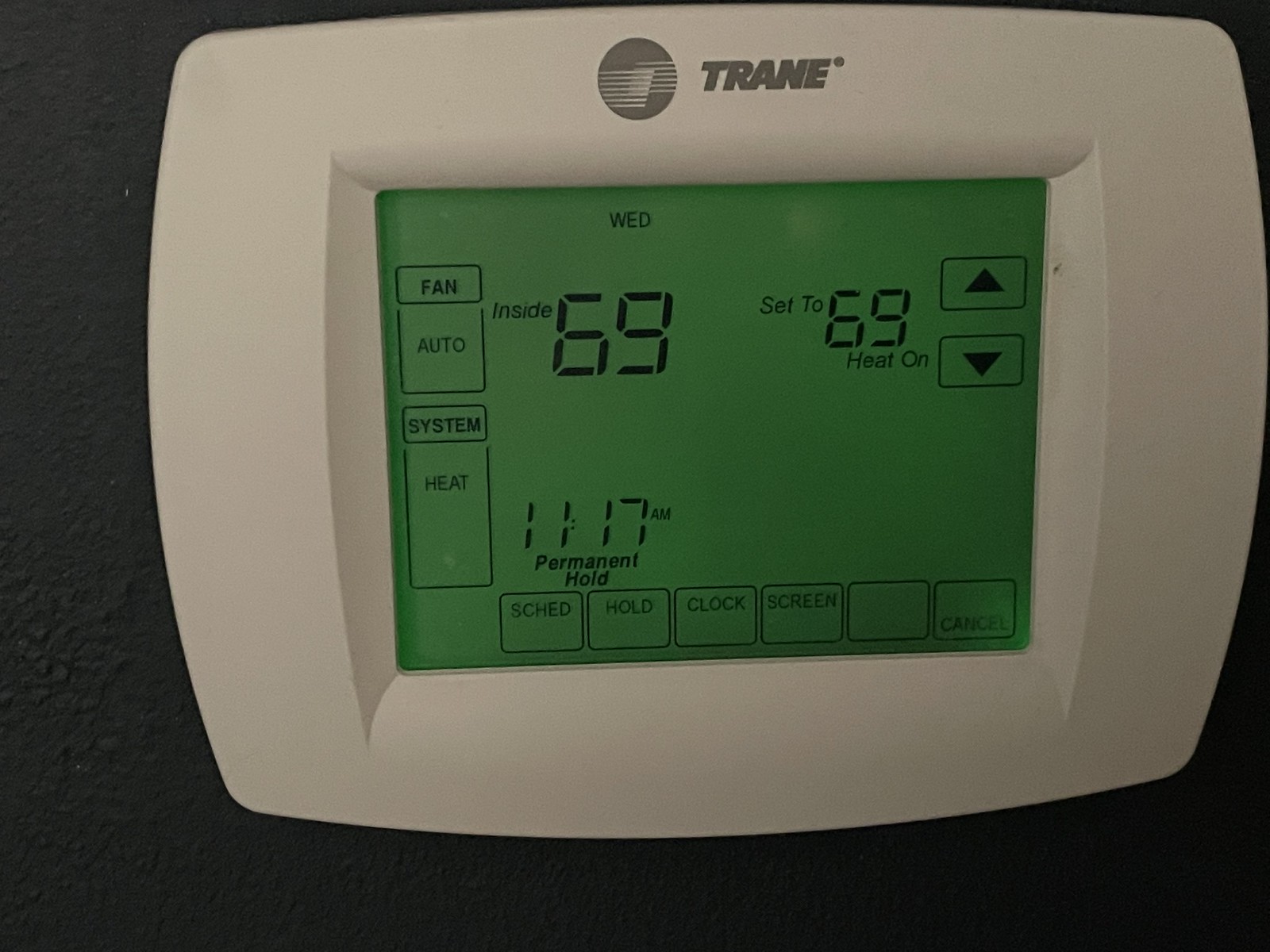The image features a white thermostat centrally mounted on a textured black wall. The wall's surface is rugged, with noticeable bumps and grooves, particularly pronounced in the bottom left corner, giving it a rough tactile quality. These textured details persist upwards, albeit less prominently, signifying deliberate design choice. Shadows obscure some of the texture near the bottom, but the pattern likely extends across the entire wall.

The thermostat itself has a modern design with rounded edges and a sleek interface. A small grey circle, intersected by lighter grey lines, houses uppercase grey letters spelling "TRANE." The device's digital display features a green backlight, showing the current indoor temperature as 69°F, matching the set temperature. The screen also indicates the system is set to "heat" mode, and the time is 11:17. Additional setting options are available for further customization.